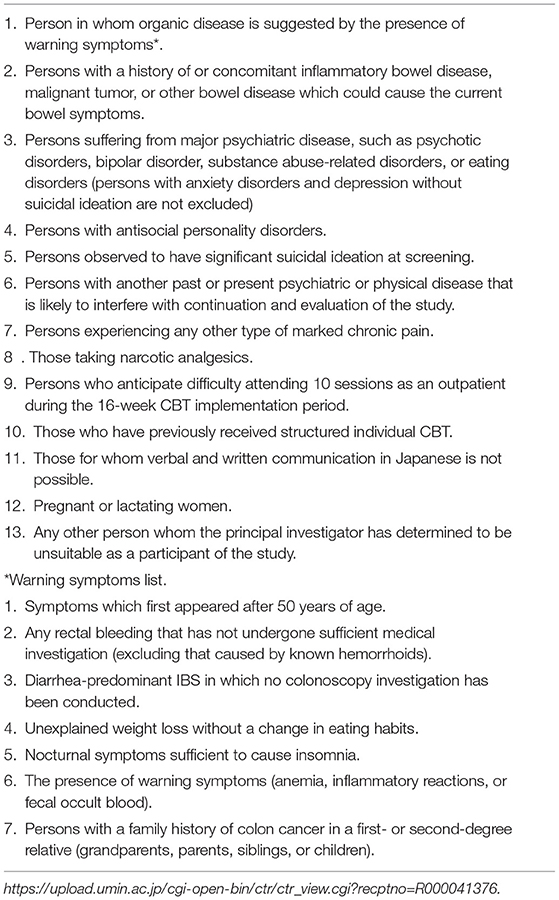The image displays a comprehensive list of exclusion criteria on a white background. A prominent black line runs horizontally across the top of the image. On the left side, the list is numbered sequentially, and to the right of each number is a detailed description of each criterion. The criteria listed from top to bottom are:

1. **Person in whom organic disease is suggested by the presence of warning symptoms.**
2. **Person with a history of or concomitant inflammatory bowel disease, malignant tumor, or other bowel diseases which could cause the current bowel symptoms.**
3. **Person suffering from major psychiatric diseases such as psychotic disorder, bipolar disorder, substance abuse-related disorders, or eating disorders. Also includes persons with anxiety disorders and depression without suicidal ideation or non-exclusionary.**
4. **Person with antisocial personality disorders.**
5. **Persons observed to have significant suicidal ideation at screening.**
6. **Persons with another present psychiatric or physical disease that is likely to interfere with the continuation and evaluation of the study.**

Each criterion is clearly outlined to ensure a meticulous assessment for appropriate study participant selection.